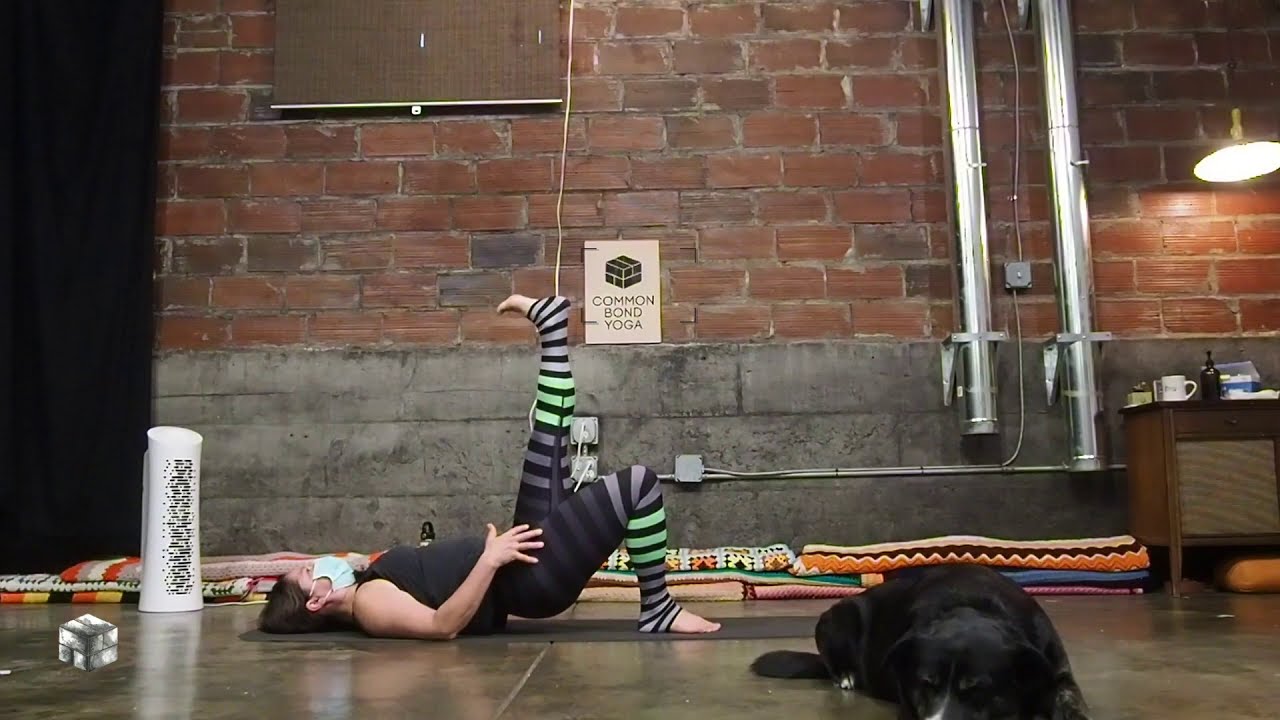In a yoga studio setting, a woman is lying on her back on a dark-colored mat placed on a tiled floor. She is positioned slightly towards the center left of the image, facing upwards. She is wearing striped leggings that transition from black and gray to green around the calf area, a black shirt, and a face mask. Her left leg is extended straight up with a yellow cord attached to it, while her right leg is bent with the foot flat on the mat. Her right hand rests on her right hip. To her right, a small black dog with white paws is lying on the floor, appearing to be resting or sleeping.

The background features a distinctive brick wall with red bricks at the top and gray concrete blocks at the bottom. To the right of the scene, there is a desk adorned with a coffee mug, a beer bottle, and a stationary lamp hanging overhead with its light on. Metal pipes are visible on the right-hand side of the wall. A sign on the brick wall reads "Common Bond Yoga" in cream-colored text, accompanied by a spherical logo. Additionally, a white object, possibly an air filter or fan, and some blankets are visible near the bottom of the wall. The entire composition of the image suggests a calm and focused environment suitable for yoga practice.